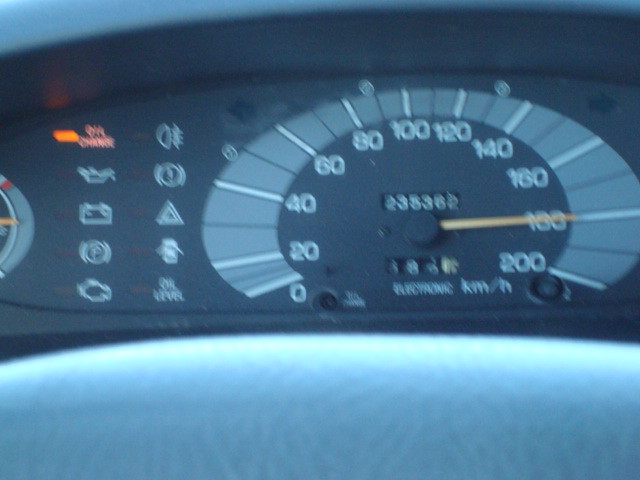This detailed color photograph captures a vehicle's speedometer and odometer. The speedometer displays speed increments from 0 to 200 kilometers per hour, marked at intervals of 20. It currently indicates a speed of 180 km/h. In the center of the image, the odometer shows a reading of 235362 kilometers. Additionally, the oil change indicator light on the top left is flashing orange, signifying that maintenance is required. The lower portion of the image is illuminated by a faint light, revealing part of the dashboard or steering wheel. This forms the entirety of the visible elements in this detailed snapshot.